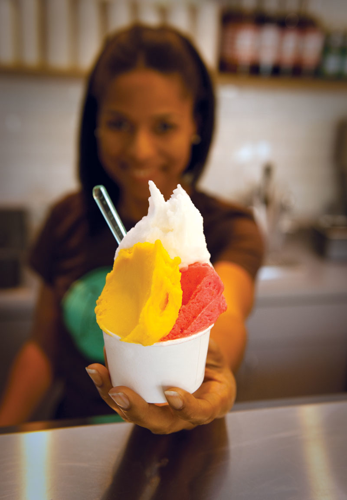In this photo, we see an African-American woman standing in an industrial kitchen setting, wearing a t-shirt with a green logo. Her hair is styled straight down and tucked back, possibly with a headband or in a ponytail. Despite her features being slightly blurry, she is visibly smiling. The main focus of the image is her hand, which is extended towards the camera, holding a white paper cup containing a trio of colorful frozen desserts—sherbet or gelato—featuring distinct yellow, red, and white scoops, with a clear plastic spoon sticking out. Her hand rests against the edge of a gray table, which is part of the kitchen setup that includes a sink, shelves with extra cups, and various other kitchen items in the background, indicating that she is preparing to hand you your order.